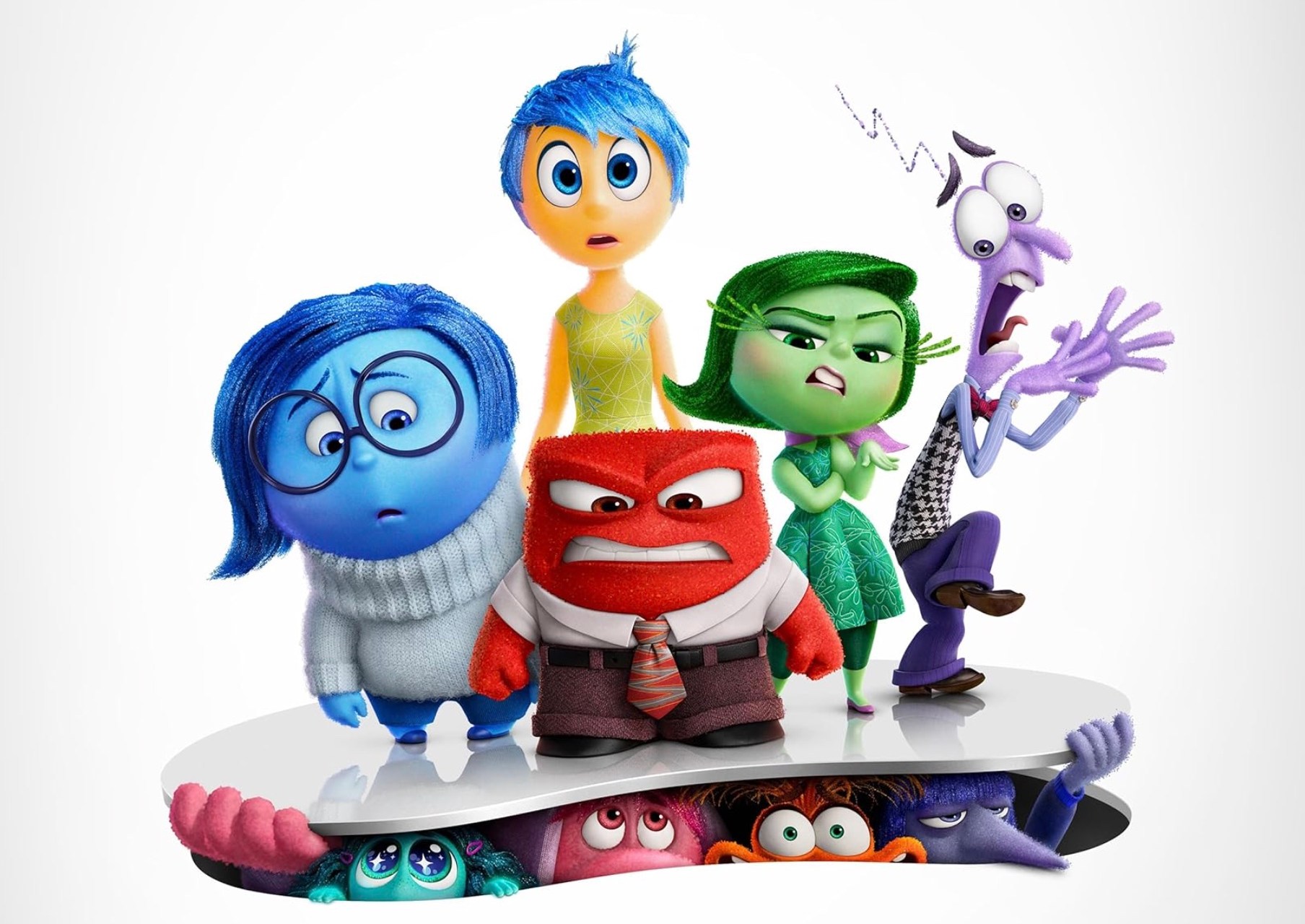The image is a rectangular frame, approximately six inches wide and four inches high, featuring characters from the Disney Pixar movie "Inside Out". The background is a subtle light gray that darkens at the corners. At the center of attention are the well-known characters from the original movie: Anger is positioned in the front center with Sadness to his left, Disgust and Fear on his right, and Joy standing slightly behind them. These characters are standing on an elevated, light gray oblong platform.

Underneath the platform, peeking curiously, are four new characters suggesting their upcoming roles in the sequel, "Inside Out 2". The leftmost figure is a blue character with just two visible eyes, followed by a large pink hand nearby. To the right, a greenish-blue character looks up gently. Next, there is a larger pink character peeping out, along with an orange character with googly eyes. On the far right, helping to support the platform, there is a skinny, purple monster-like figure with a distinct carrot-shaped nose.

The composition reflects a dynamic scene where the original characters from the first movie appear concerned or curious about the newcomers emerging from beneath.